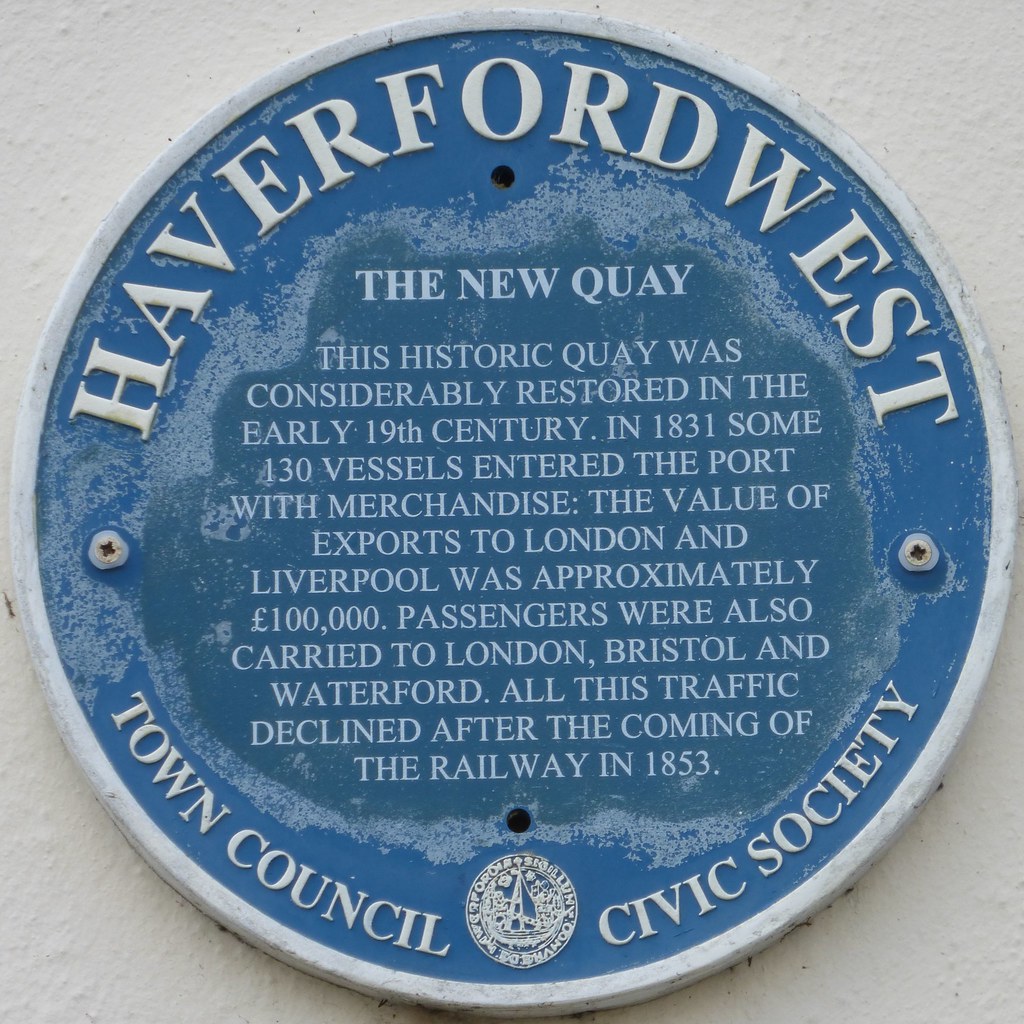The image features a weathered, blue circular plaque bordered by a silver bezel, likely positioned at the entrance or base of a tourist attraction. The top of the plaque displays "Haverford West" in prominent white lettering, while the bottom reads "Town Council Civic Society." Centrally, the plaque is titled "The New Quay" and provides historical information: "This historic quay was considerably restored in the early 19th century. In 1831, some 130 vessels entered the port with merchandise. The value of exports to London and Liverpool was approximately £100,000. Passengers were also carried to London, Bristol, and Waterford, and all this traffic declined after the coming of the railway in 1853." The font color is mainly white, against the faded blue background, with the inscription highlighting the quay's significance and historical details.